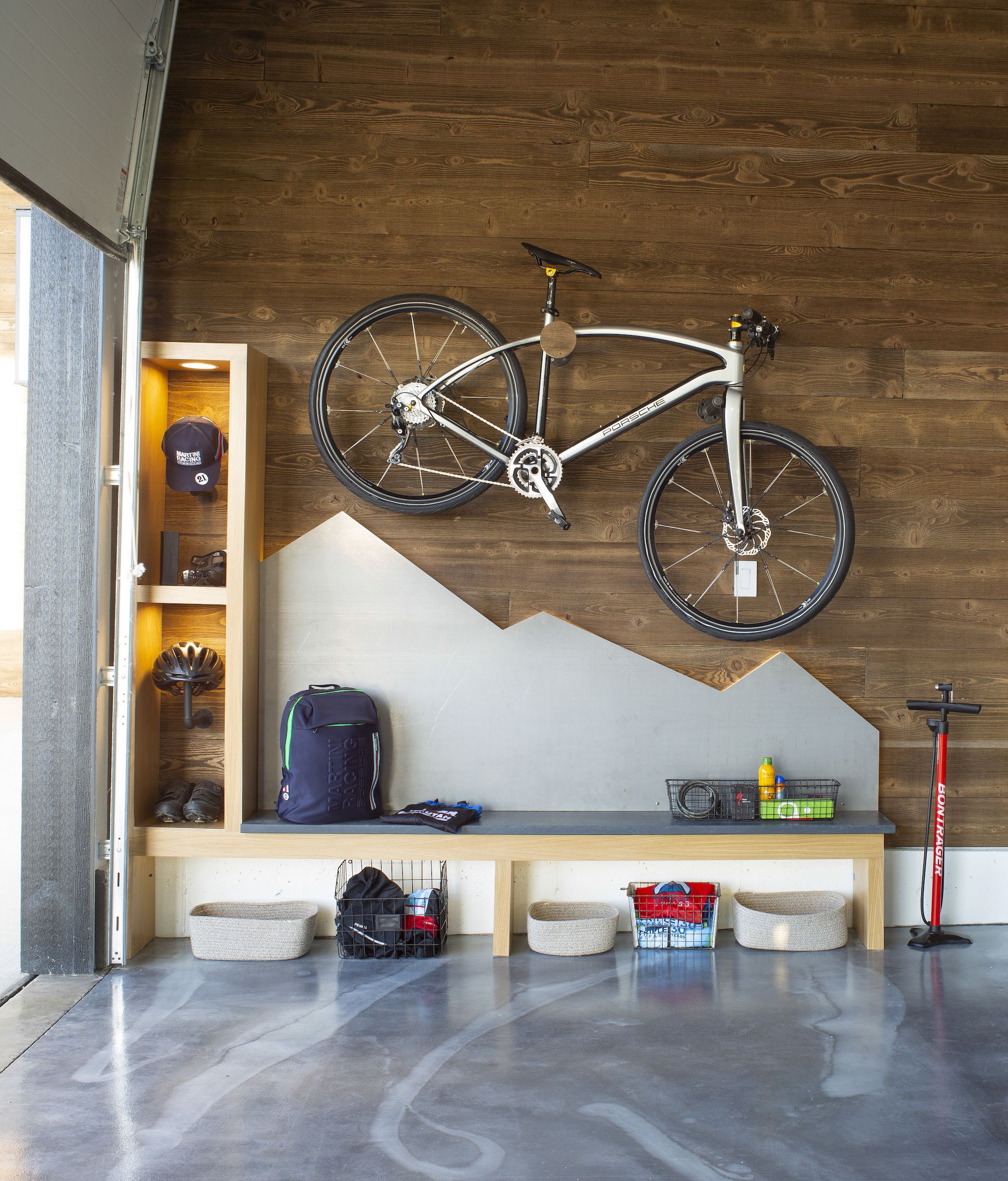The image depicts the interior of what appears to be a large, well-lit space, potentially a garage or a storage area. The main feature is a mountain bike, which is mounted on a wood-paneled wall, giving the impression of descending a set of stylized, light-gray mountains painted below it. The bike itself is silver and appears to be relatively new. 

Adjacent to the bike, on the left, is a shelf containing various items including hats, lights, shoes, and helmets. This shelf seamlessly transitions into a gray wooden bench that supports a blue backpack and a basket holding bottles. Below the bench are additional baskets, some woven and some wire, filled with miscellaneous items. To the right of the bench, there's a bike tire pump positioned in the lower corner.

The floor of the room is smooth and shiny, made of a sleek gray material, which reflects the ample daylight streaming in, likely from a large bay door visible on the left side of the image. The space is open and tall, enhancing the feeling of spaciousness and organization within this functional yet aesthetically pleasing interior.